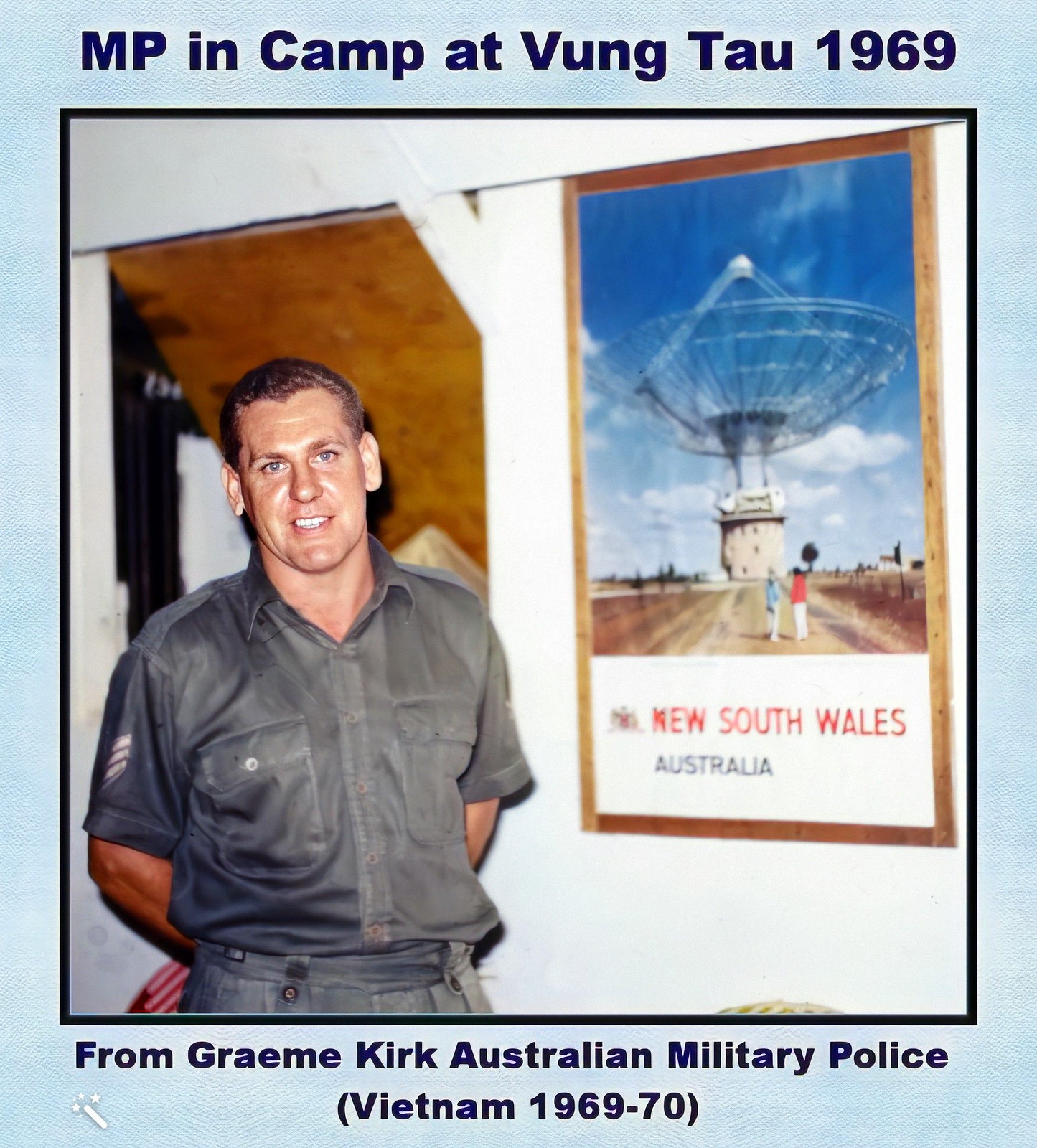The image features a carefully framed photograph with a light blue header and footer, and matching side borders that are narrower. These borders are further accentuated by a thin black pinstripe encasing the photo. At the top in bold navy blue or black print, the header reads "MP in camp at Vung Tau 1969," though “Vung Tau” is misspelled as “Bung-Tau.” The footer states in the same font and color, "from Graeme Kirk, Australian Military Police (Vietnam 1969-70)."

Centrally, the photograph showcases a Caucasian man in uniform standing to the left with his hands behind his back, gazing directly at the camera. He has short, finely trimmed brown hair, appears to be in his mid-40s to early 50s, and has light-colored eyes. Behind him is a white wall adorned with a large poster on the right side that reads "New South Wales, Australia." The poster features two people in front of a massive satellite antenna, likely related to deep space communications, similar to those used by NASA's Jet Propulsion Laboratory.